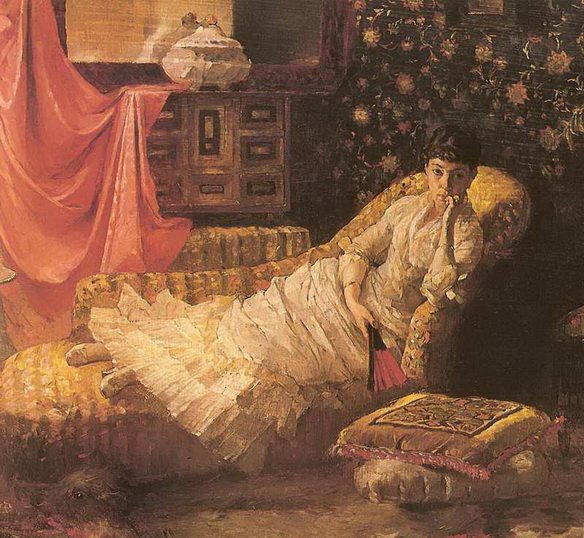The painting presents a dark and somber scene featuring a woman bathed in an almost melancholic atmosphere. She is centrally seated on a yellow-seated cushion of a chaise lounge, her dark hair styled up elegantly. She wears an elaborate, lacy white gown and holds a small, striking fan that is black and red in her right hand. Nearby, on the floor, lie two intricately designed pillows in shades of yellow and red. 

Behind her, a rich, black floral print wall adds depth and complexity to the composition, with a mirror positioned at the top left, reflecting parts of the scene. A red draped cloth cascades over a visible bureau with drawers, upon which sits a white pottery or jewelry box, adding a touch of antiquity and intrigue. The scene is completed with a glimpse of a dog at the bottom left corner and a hint of a carpet underfoot. The overall style of the painting, likely an oil painting, effectively captures the viewer’s attention with its detailed, layered elements, and the woman’s deep gaze that seems to pierce through the canvas.